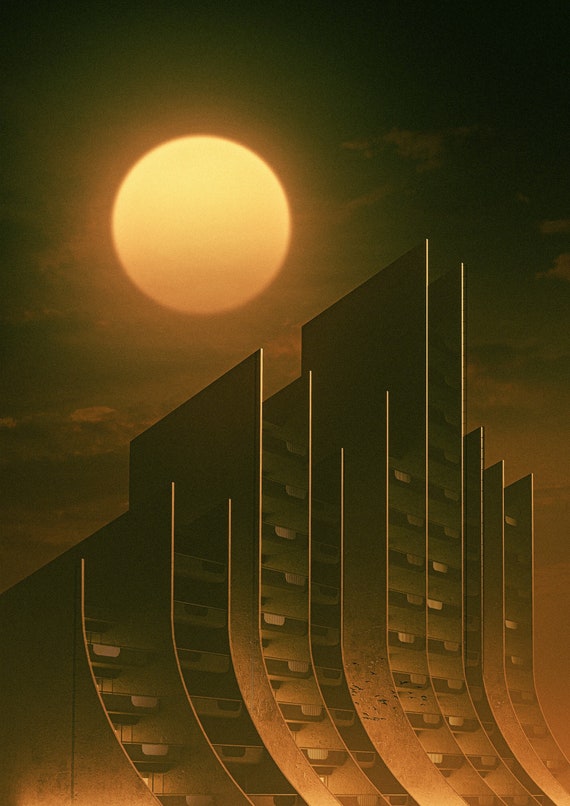This image depicts a surreal painting or drawing set against an almost black, nighttime sky. Dominating the upper left corner is a large, yellowish, slightly glowing circle that resembles a full moon, lending an otherworldly atmosphere to the scene. Below this, a series of futuristic, architectural buildings rise from the bottom left towards the right. These structures are composed of long, thin, metal-like columns that curve upwards with a sweeping gesture, giving them a dynamic and angular appearance. The buildings, varying in height, exhibit a sepia or brownish tone, with deep shadows enhancing their intricate details. Some sections of the structures are connected by small stairs or steps that ascend through the middle. The overall composition, with its contrasting yellowish and dark hues, evokes a sense of mystery and industrial elegance.